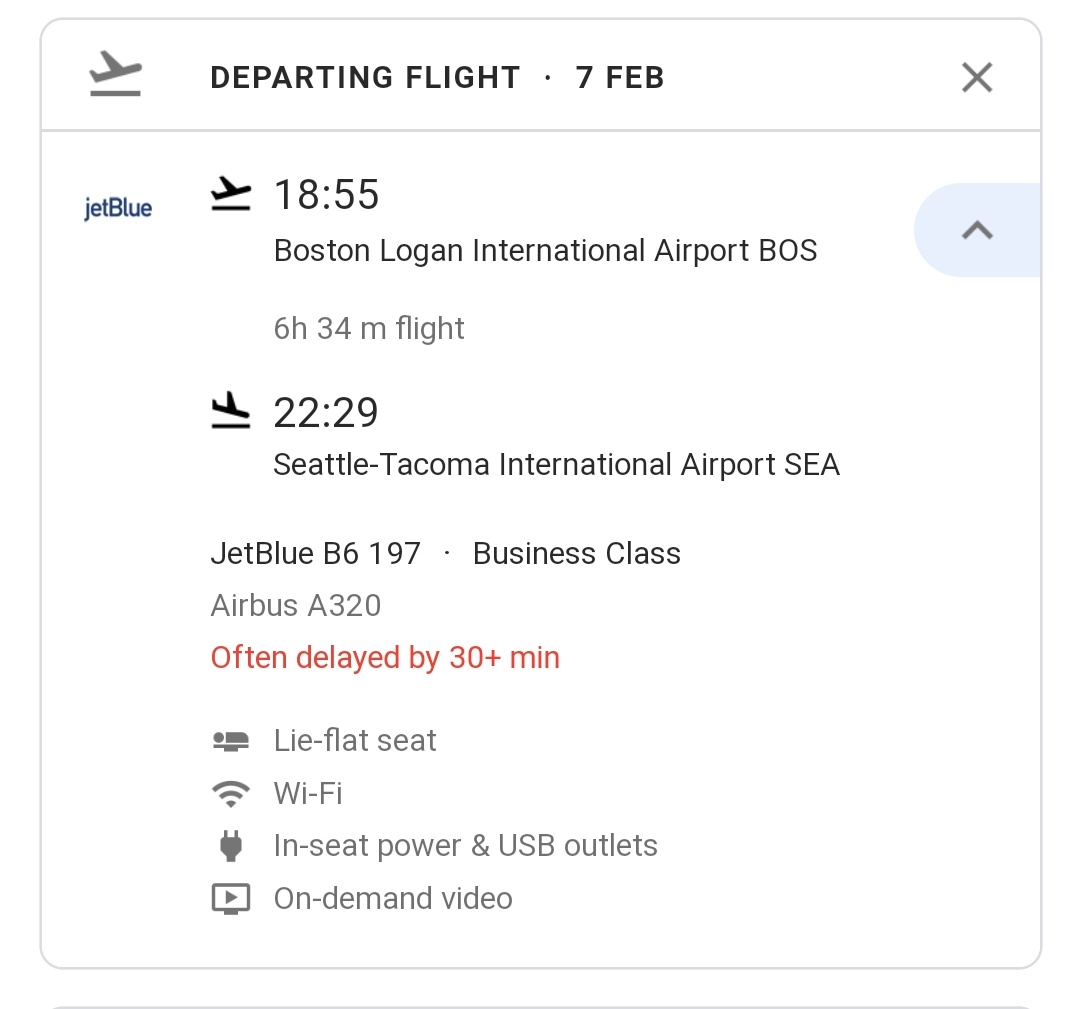This image is a detailed smartphone screenshot displaying information for a departing JetBlue flight on February 7th. At the top, there is an airplane taking off icon alongside the text "Departing Flight - 7 FEB," with a closeout 'X' to the right.

The next section includes the JetBlue logo and states the airline's name. This is followed by another airplane taking off icon and the departure time of 18:55 from Boston Logan International Airport (BOS). The duration of the flight is noted as 6 hours and 34 minutes.

Further down, an airplane landing icon is present next to the arrival time of 22:29 at Seattle-Tacoma International Airport (SEA). 

Additional flight details include:
- Airline: JetBlue
- Flight Number: B6197
- Class: Business Class
- Aircraft: Airbus A320
- Note: Often delayed by 30+ minutes

Amenities indicated in the display are:
- Lie-flat seat
- Wi-Fi availability
- In-seat power (NC power and USB outlets)
- On-demand video access

The entire section can be collapsed using a drop-down arrow to condense the information.